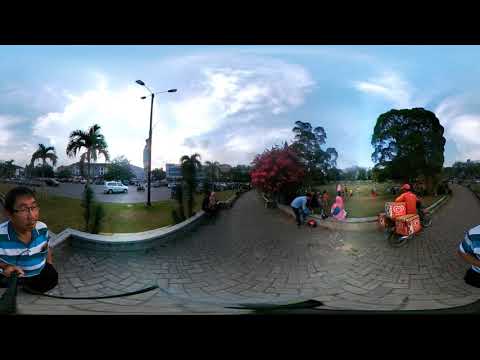In this vibrant, daytime outdoor scene, we find ourselves in a bustling public park. The foreground is accentuated by a gray stone brick path, where various individuals are engaged in their leisure activities. To the left, a man in a blue and white striped shirt and dark pants, wearing black glasses, is holding a selfie stick, suggesting a moment of personal snapshot. Nearby, a lady in a blue shirt and pants rummages through her purse, possibly to buy ice cream for a little girl dressed in pink from an orange-clad ice cream vendor on a bicycle with matching orange coolers.

The background reveals a harmonious blend of nature and urban life. Towering palm trees with brown trunks and green foliage, along with other lush green trees, frame the scene. A bush with reddish or pink flowers adds a splash of color to the verdant surroundings. Gray benches and ledges line the walkway, providing places to rest. Beyond these, gray apartment buildings loom subtly, indicating the city’s proximity.

A mix of people stroll along the path, dressed in an array of colorful clothing, creating a lively atmosphere. The park is bordered by grassy areas and a parking lot filled with various vehicles, including a white van, hinting at accessibility and convenience. The sky above is a serene blue, adorned with feathery white clouds, adding to the picturesque quality of this park scene where urban and natural elements coalesce seamlessly.